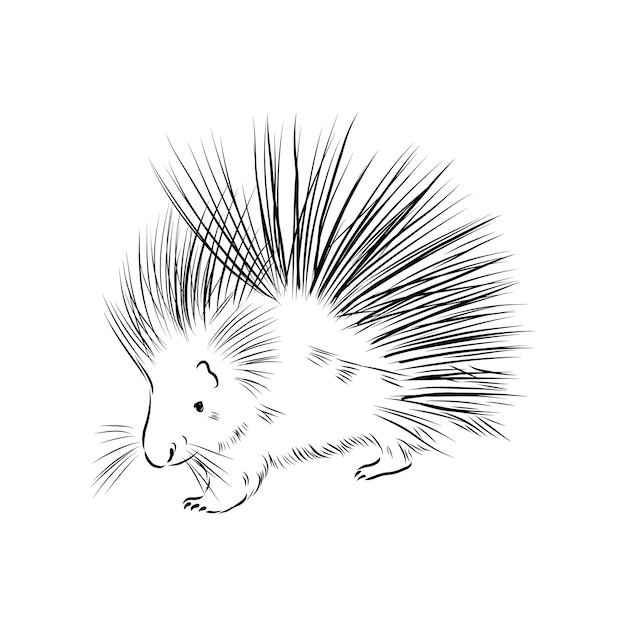This is a minimalist, black and white sketch drawing of a porcupine, featuring no border or text. The porcupine appears in profile, facing towards the lower left. It is drawn in a style that resembles a pencil sketch or graphic print, characterized by its simplicity and use of lines. The background is entirely white, blending into the body of the porcupine which also predominantly remains white, with the exception of some defining features. 

The porcupine's head is positioned on the left side, showcasing a small circle for the eye, accompanied by texture lines, and a curved line delineating the nose. Whiskers extend outward, with five or six longer lines drawn on each side. The small, pointed ear is visible near the top of the head. The paws and legs are also depicted, with small curved lines indicating the nails. 

The spikes begin at medium length on top of the head and grow longer as they cascade down the back, nearly doubling in length before tapering slightly at the tail end. These spikes, drawn with black lines, point in various directions, predominantly from the upper left to the lower right, creating a sense of dynamic motion and texture.